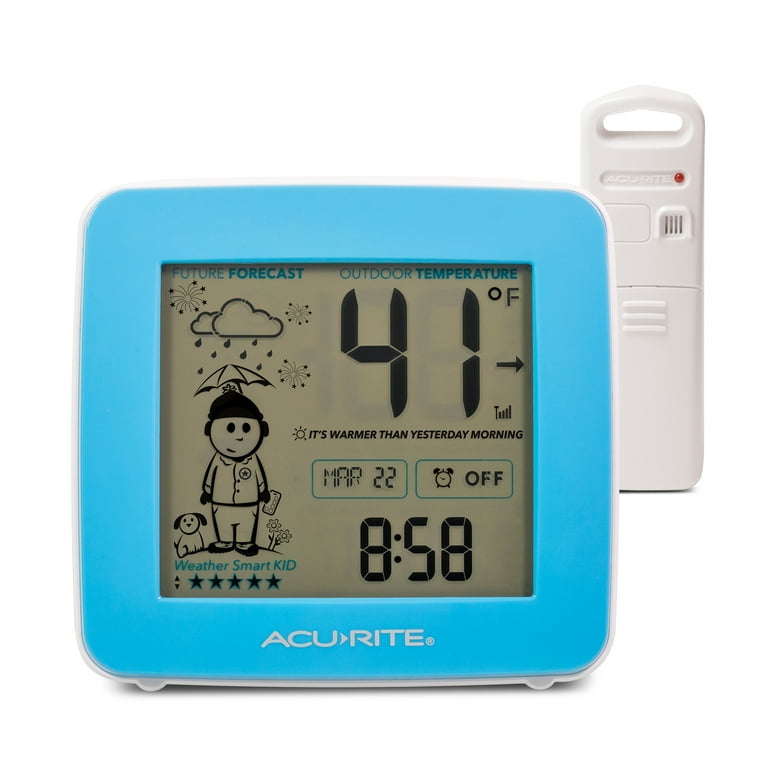This photograph features a compact, square-shaped digital device, likely a combination digital thermometer and thermostat for home use, with precise detailing on a plain white background. The focal point is the AcuRite device, approximately four inches by four inches, encased in a thin white plastic frame with rounded feet at the bottom. The front of the screen is bordered by a light blue frame about half an inch thick. Dominating the screen, in light brown, is a detailed display.

At the top left, "Future Forecast" is written in blue, above a vibrant illustration of a person dressed in cold-weather clothing standing under an umbrella with a dog beside them. Rain is depicted falling from a cloud over the umbrella, with a festive touch of fireworks in the background. Immediately below, in blue, "Weather Smart Kid" is labeled, accompanied by five stars.

On the right side of the screen, the words "Outdoor Temperature" are printed in blue above a black digital display reading "41°F." Beneath, additional text states, "It's warmer than yesterday morning." The date, March 22nd, is shown in two black-printed ovals with blue outlines, and the time "8:58" appears below, indicating the alarm is off.

In the background, a small white remote control for the device is visible, featuring a single button, a speaker, and a red light, with recessed text indicating "AcuRite." The comprehensive information and clear visual cues make this AcuRite device an informative and charming gadget for monitoring weather conditions at home.